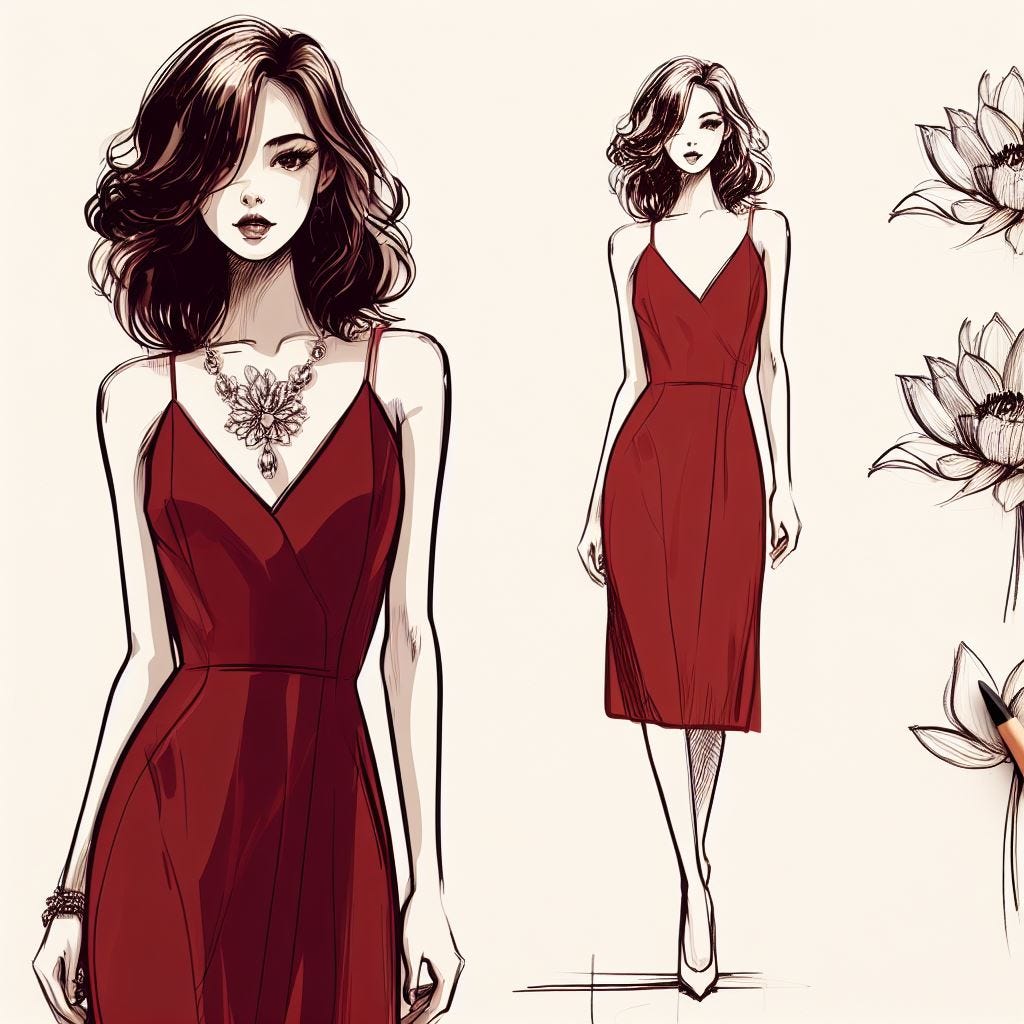The image is an illustration resembling concept art, envisioning a cover for a fashion magazine, likely by a women's clothing designer. It features a model depicted twice, once in a close-up and once in a full-body view. The model, a slim woman with long, slightly curly light brown hair that covers her right eye, is adorned in a elegant red cocktail dress that extends just below her knees. The dress is cinched at the waist, has a V-shaped neckline, and delicate spaghetti straps. In the close-up, the model showcases a large, elaborate floral necklace, possibly made of metal or adorned with diamonds, and wears a bracelet on her right wrist. This close-up possibly reaches until mid-thigh. In the full-body view, she's seen wearing high heels. Surrounding the main illustrations are sketched flowers on the right side of the image, and a sharpened pencil rests atop one flower, emphasizing the sketch’s artistic theme.